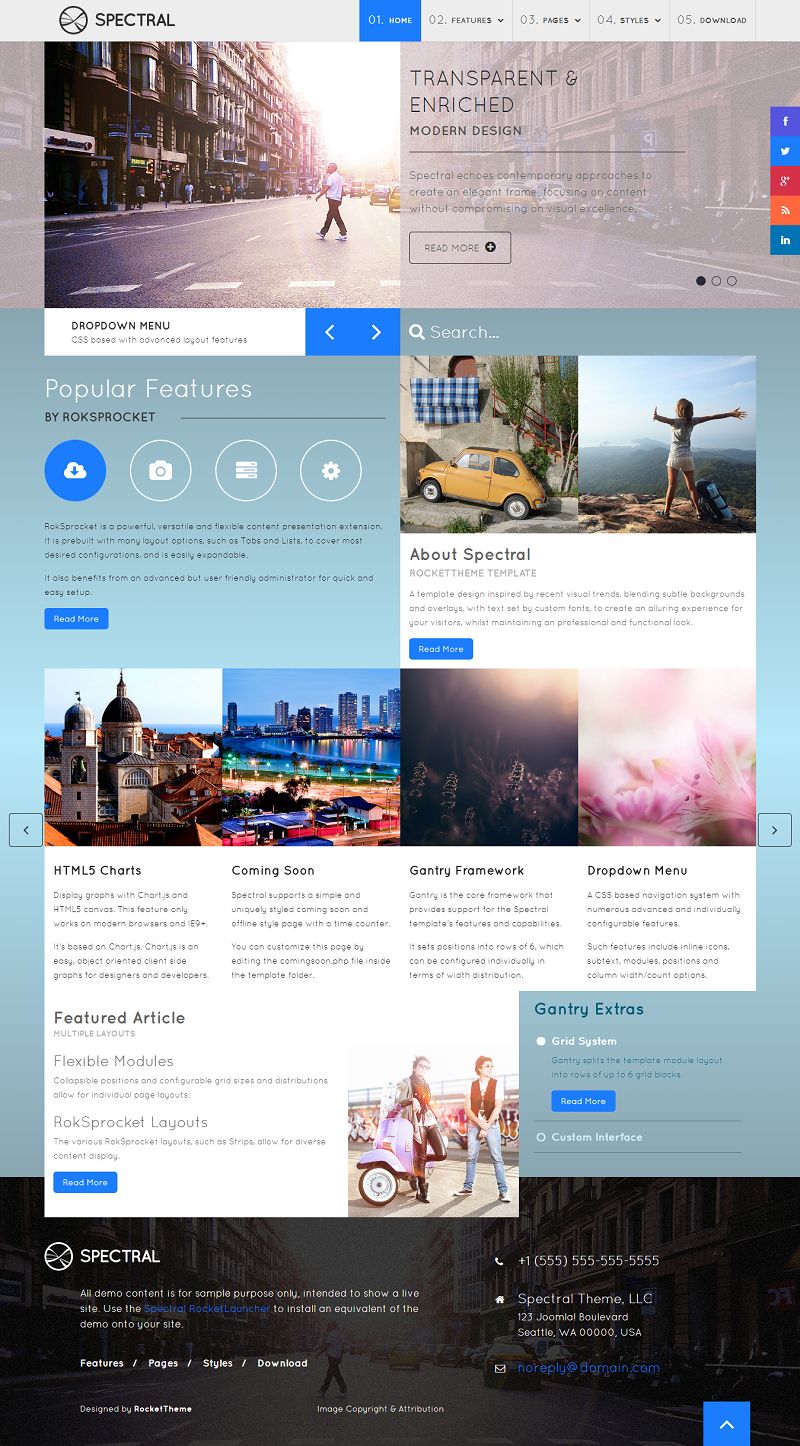Homepage of the Spectral Website

The homepage of the Spectral website features a meticulously organized layout. 

In the top-left corner, there is a distinctive logo comprised of a circle with two lines intersecting inside it, rendered in fine detail. Adjacent to the logo is the word "SPECTRAL" written boldly in black, all capitalized. 

On the far right of the page, blurred statistics are visible.

Beneath the header, various images are neatly arranged. 

In the top-left section, an image depicts a man walking down a busy, multi-lane city street. Cars are parked to the right, while towering multi-story buildings line the left. Below the image, the phrase "TRANSPARENT AND ENRICHED MODERN DESIGN" is prominently displayed.

Below this, a section titled "POPULAR FEATURES" by Rock Sprocket showcases four icons: a gear symbol, a camera, a download icon, and a file icon.

To the right of the feature list, another visual element includes an image of a small yellow car and a woman standing on a cliff with her arms outstretched, facing the sun. This section is labeled "ABOUT SPECIAL."

Additional images on the page capture a variety of scenes, including old buildings in a city, modern architectural structures, and picturesque natural landscapes.

At the bottom of the page, a blurred section contains contact information, including telephone numbers and addresses.

The footer also announces a "COMING SOON" section related to a gantry framework drop-down menu.